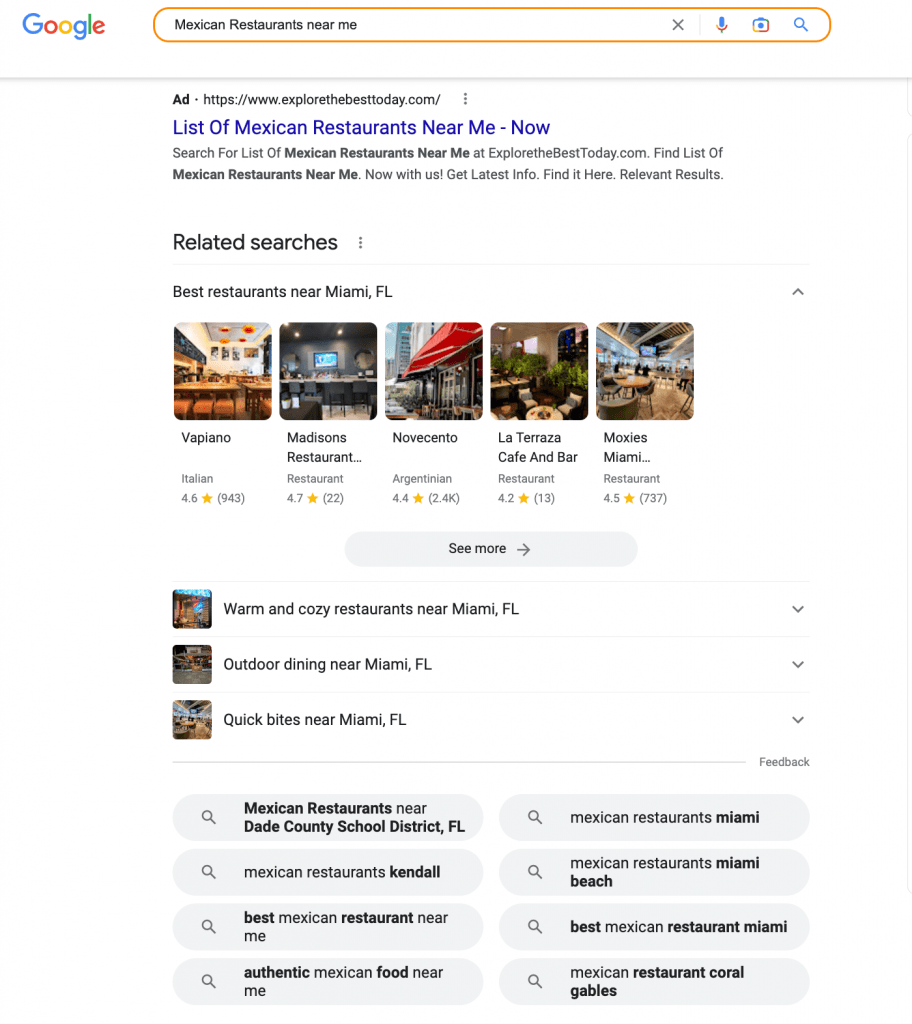The image shows a Google search page with location services enabled, displaying results for "Mexican restaurants near me." The top search result, marked as an ad, directs users to "explorethebesttoday.com" for a comprehensive list of Mexican restaurants. The site promises up-to-date information with a call to "search for a list of American restaurants near me" and a clickable button labeled "relevant results." The search appears to be conducted near Miami, Florida, as indicated by the header "best restaurants near Miami, Florida."

Several restaurant listings are presented, each with accompanying images and ratings:
1. **Vapiano** - Rated 4.6 stars
2. **Madison's Restaurant** - Rated 4.7 stars
3. **Novecento (Argentinian)** - Rated 4 stars
4. **La Terraza Cafe and Bar** - Rated 4.2 stars
5. **Moxie's near Miami** - Rated 4.5 stars with a notable number of reviews

The search results include options for other restaurants and areas, suggesting ease of finding a suitable Mexican restaurant nearby.